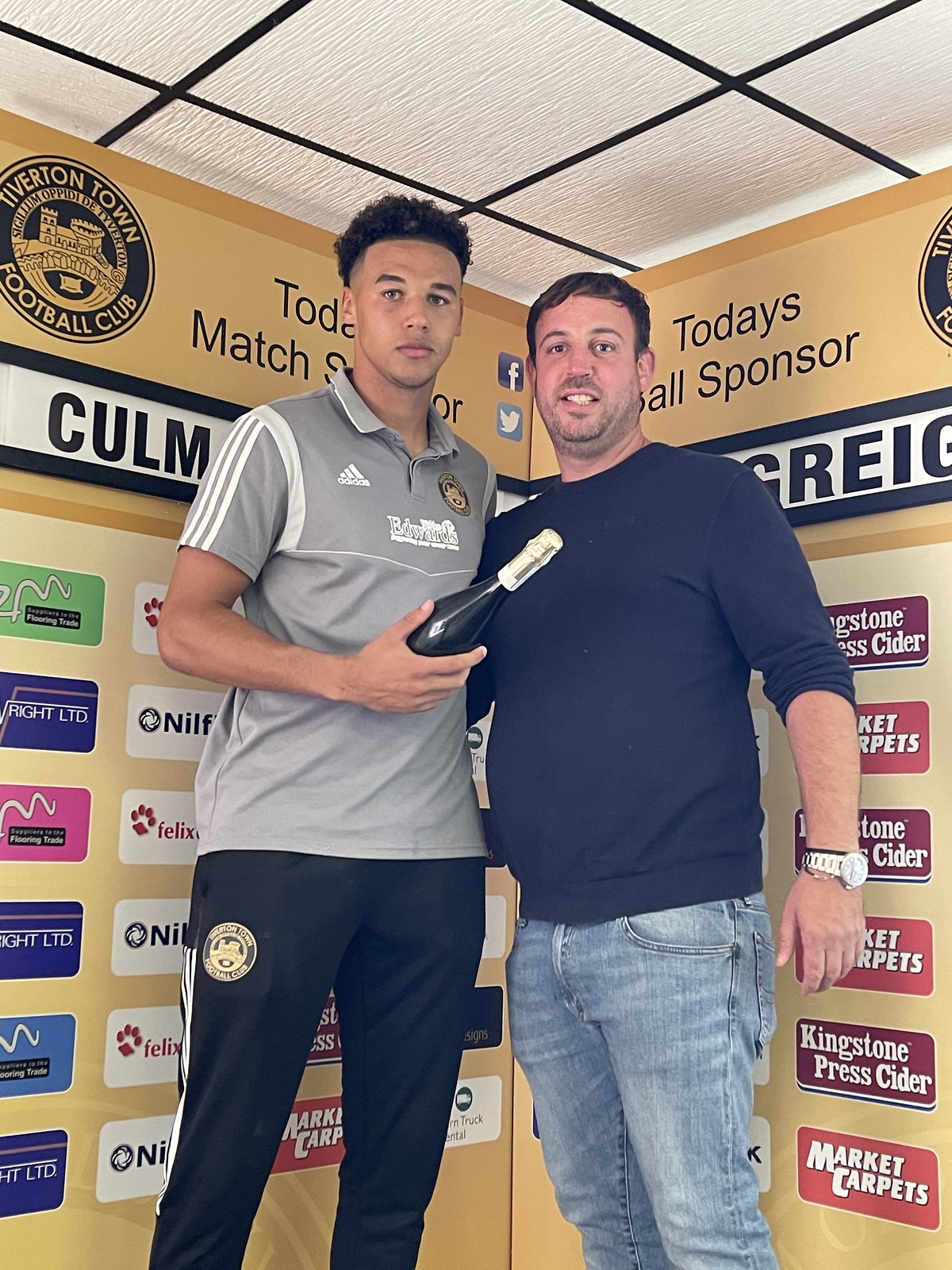Standing in front of a golden yellow advertisement-covered sign, two men pose side-by-side, slightly off-center in a narrow space that appears to be the corner of a small building or tent. The sign, bent at a corner, is topped with a black and gold circle logo reading "Tiverton Town Football Club" and has several sponsor logos, including partially visible names like "Felix" and "Nilf." The ceiling above them features white textured tiles bordered by black lines. 

The man on the left, who could be an athlete, is taller with light brown skin and curly black hair. He's wearing a short-sleeved gray and white Adidas shirt, black sweatpants, and is holding a black bottle in his right hand. The man on the right, likely older with a stubble beard, is dressed in a long-sleeved blue shirt, light blue jeans, and a watch on his left wrist. The backdrop's multiple logos and signs around them, including social media icons for Facebook and Twitter, suggest a promotional or sponsorship event related to a football match.